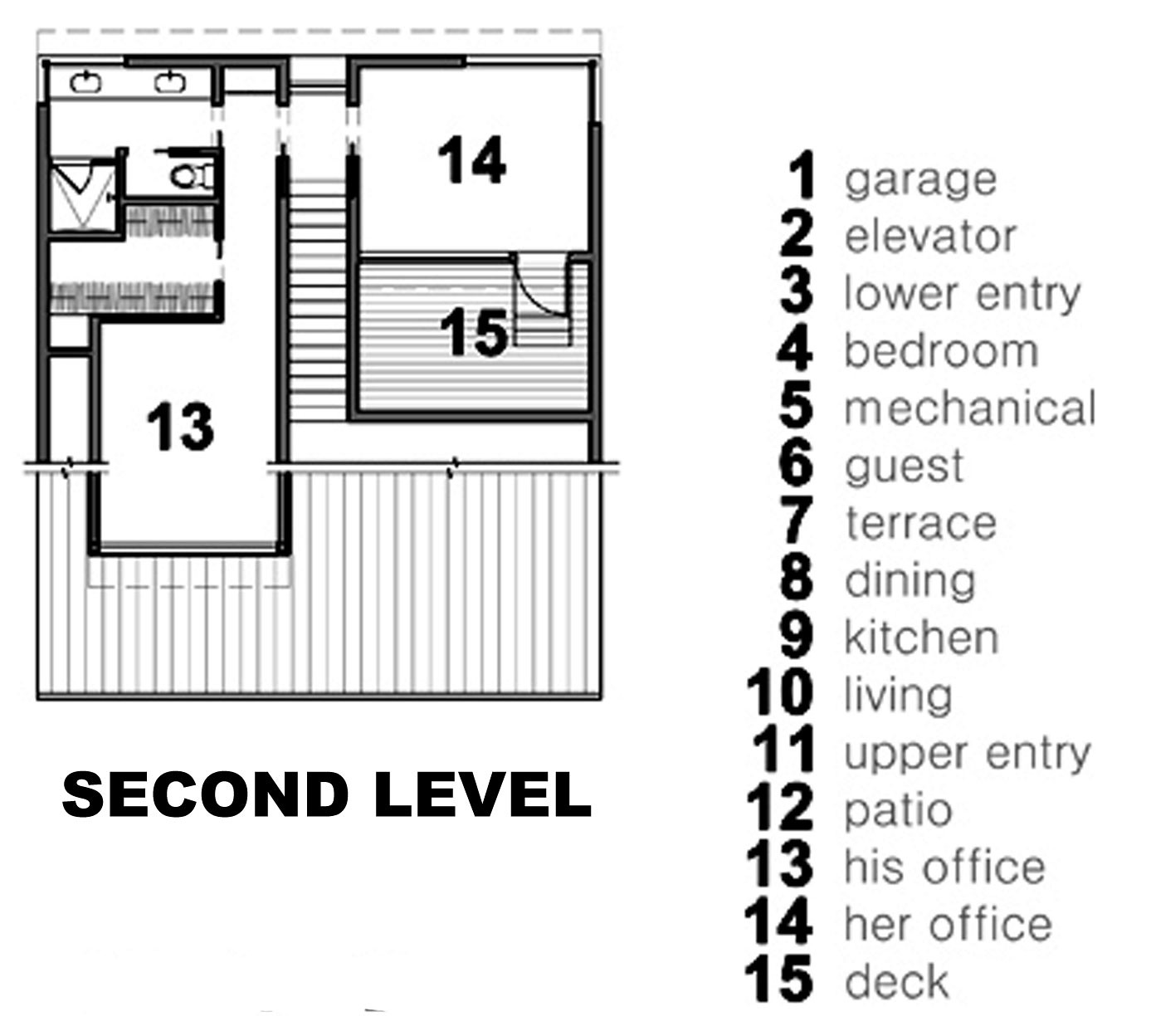This image depicts a detailed sketch of a second-level floor plan, as indicated by the black text reading "second level" below the plan. The floor plan includes various identifiable features such as stairs and a bathroom. On the right side of the image, there is a legend listed from numbers 1 to 15 in bold black text, with each number corresponding to a specific area of the floor plan, denoted in light gray text. The legend includes the following labels: 1) Garage, 2) Elevator, 3) Lower Entry, 4) Bedroom, 5) Mechanical, 6) Guest, 7) Terrace, 8) Dining, 9) Kitchen, 10) Living, 11) Upper Entry, 12) Patio, 13) His Office, 14) Her Office, and 15) Deck. However, only numbers 13, 14, and 15, which correspond to 'His Office,' 'Her Office,' and 'Deck,' respectively, are visible on the actual floor plan.